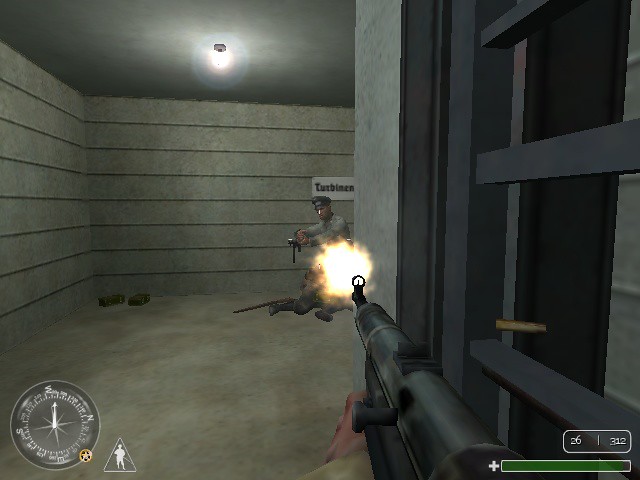The image is a screenshot from a video game, depicting a tense scene inside a dimly-lit bunker or tunnel. The environment is constructed from light-colored cement, with darker gray ceilings and patches of light-colored dirt scattered across the floor. The player's perspective showcases a long firearm with a small scope, held by a character wearing a tan shirt, revealing a white hand.

On the right side, a dark gray structure resembling a door or window is partially visible. Flames burst from the end of the player's gun, illuminating the legs of a fallen individual sprawled on the floor, suggesting that the player may have just shot them. Nearby, a discarded gun lies on the ground.

Slightly behind this fallen figure, another man is crouched, dressed in a dirty shirt and wearing a hat reminiscent of a police cap. This light-skinned character is also armed, heightening the sense of danger.

The game interface elements are visible as well. On the bottom left corner, there is a compass, along with icons of a small person, a triangle, and a star. The bottom right corner displays the number "26," a vertical line, the numbers "312," and a nearly full power bar, conveying critical gameplay information.